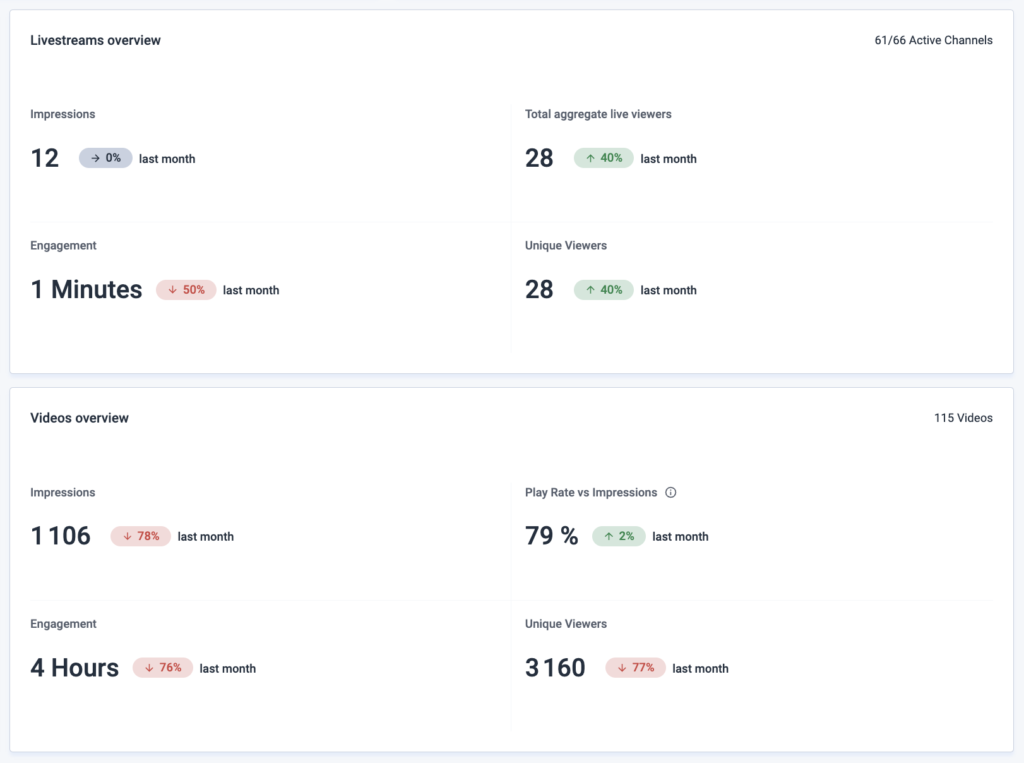The image is a detailed screenshot of an overview page for a fan page, divided into two main sections.

The top section on the left is titled "Live Streams Overview." It contains the following statistics:
- Impressions: 12 (no change from last month).
- Total Aggregate Live Viewers: 28 (up 40% from last month).
- Engagement: 1 minute (down 50% from last month).
- Unique Viewers: 28 (up 40% from last month).

To the right of this section, it states, "61 out of 66 active channels."

The bottom section on the left is titled "Videos Overview." It contains the following statistics:
- Total Videos: 115.
- Impressions: 1,106 (down 78% from last month).
- Engagement: 4 hours (down 76% from last month).
- Play Rate vs Impressions: 79% (up 2% from last month).
- Unique Viewers: 3,160 (down 77% from last month).

In each section, metrics that have decreased are indicated with red-colored ovals and numbers, while metrics that have increased are highlighted with green-colored ovals and numbers.